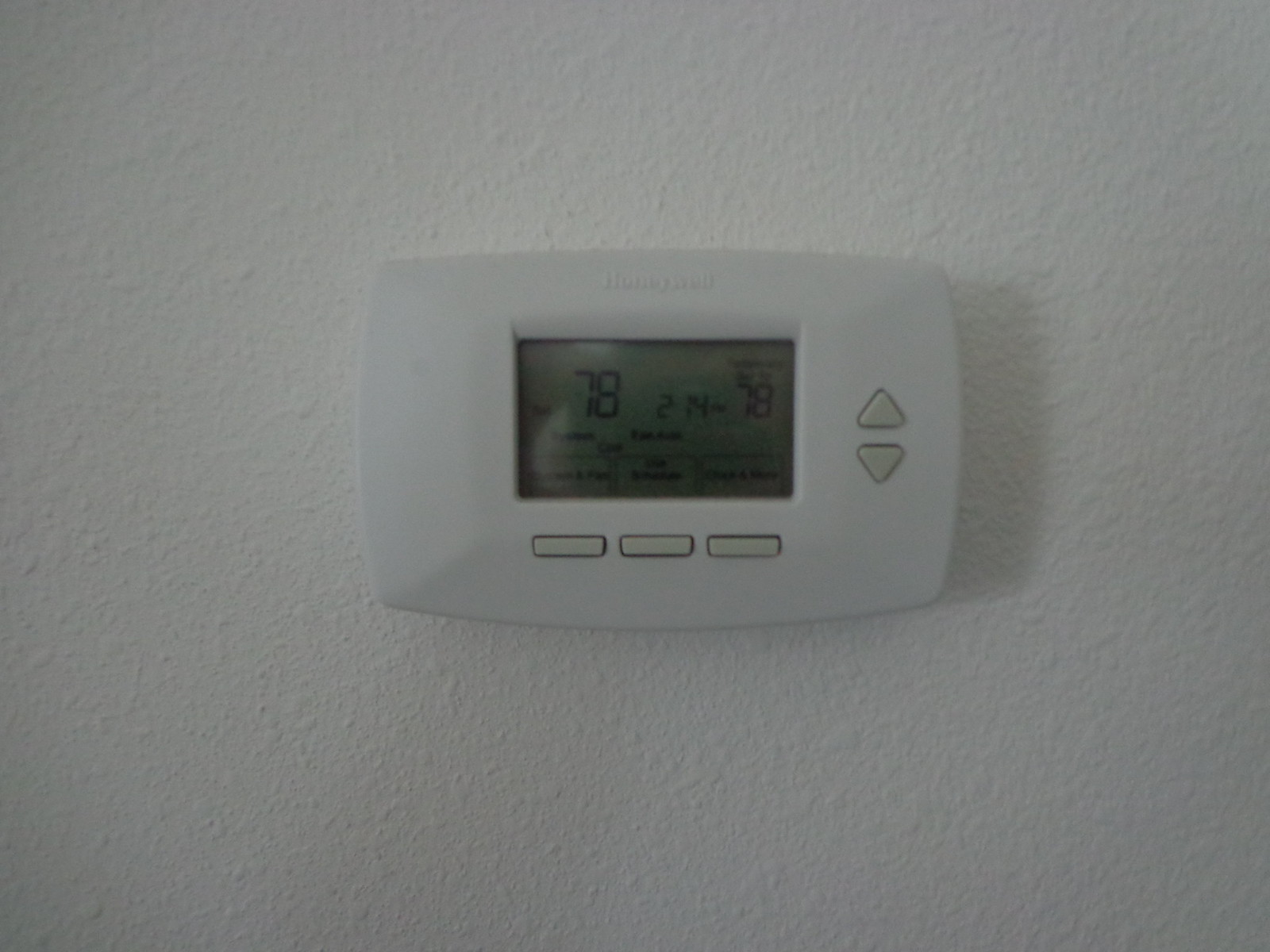The image showcases a white wall with a textured surface, upon which a sleek, smooth white thermostat is mounted. The thermostat features a digital screen displaying the temperature as 78 degrees, along with a time reading of 2:14 PM. There are additional words on the screen that are not legible in the image. Directly beneath the screen, there are three small rectangular buttons lined up horizontally. To the right of the screen, there are two vertical arrow buttons; the top arrow points upwards, and the bottom arrow points downwards. These buttons are used to adjust the thermostat settings, allowing the user to switch between air conditioning and heating modes and set the desired room temperature. The upward arrow increases the temperature setting, while the downward arrow decreases it.